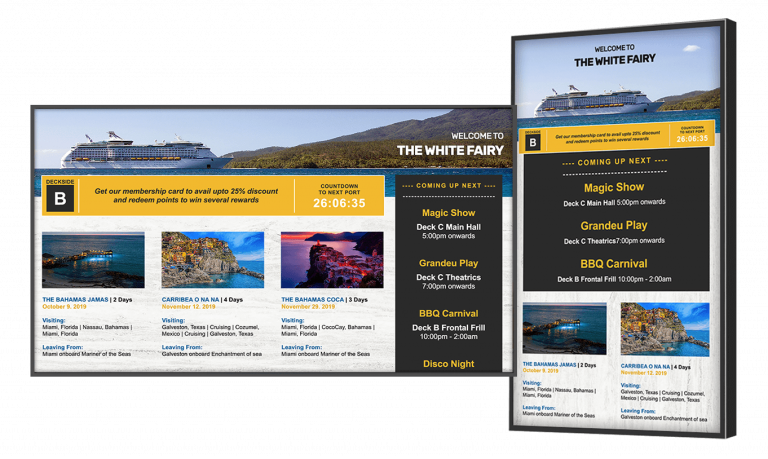In this image, there are two devices with screens, one positioned horizontally and the other vertically. The horizontal screen displays various announcements and offers related to the vessel named "White Ferry." Notably, it promotes a membership card that provides up to a 25% discount and the opportunity to earn points for rewards. There is also a countdown indicating that the next port arrival is in 26 hours, 6 minutes, and 5 seconds. The upcoming events are highlighted: a Magic Show at 5 PM in Deck C’s main hall, a theatrical performance of Brandew Play at 7 PM in Deck C, and a BBQ Carnival at Deck B’s front from 10 PM to 2 AM, offering a discount. Additionally, the screen mentions the arrival of the "Bahamas Jammers," who are visiting today and leaving from Colosia. The description includes the colors black, yellow, and brown associated with the Bahamas Jammers. The vertical screen prominently features an image of a majestic cruise liner, likely the White Ferry itself.